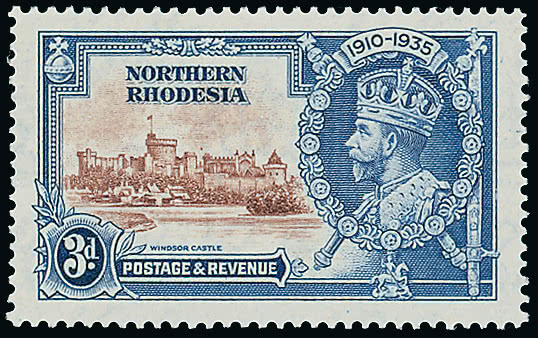This is a detailed photograph of a rectangular postage stamp from Northern Rhodesia, set against a black background. The stamp itself features a white border designed with scalloped edges. Dominating the right side of the stamp is a central portrait of a king in profile, who is most likely of white complexion, adorned with a cracked crown. The king has a beard and mustache and his headshot is encircled by an oval ribbon design. Above the portrait are the years "1910-1935," signifying a commemorative period. To the left of the portrait, the stamp reads "Northern Rhodesia," and below in a tan section is an illustration of Windsor Castle in a darker tan hue. Beneath this image is a dark blue band with the inscription "Windsor Castle" in blue and "Postage and Revenue" in white. Additionally, there is a shield design featuring the text "3D." The top part of the stamp includes motifs resembling leaves and a ball topped with a cross, along with a circular emblem containing crossed swords and a flower garland. At the bottom center, underneath the portrait, there is also a depiction of a person on a horse.